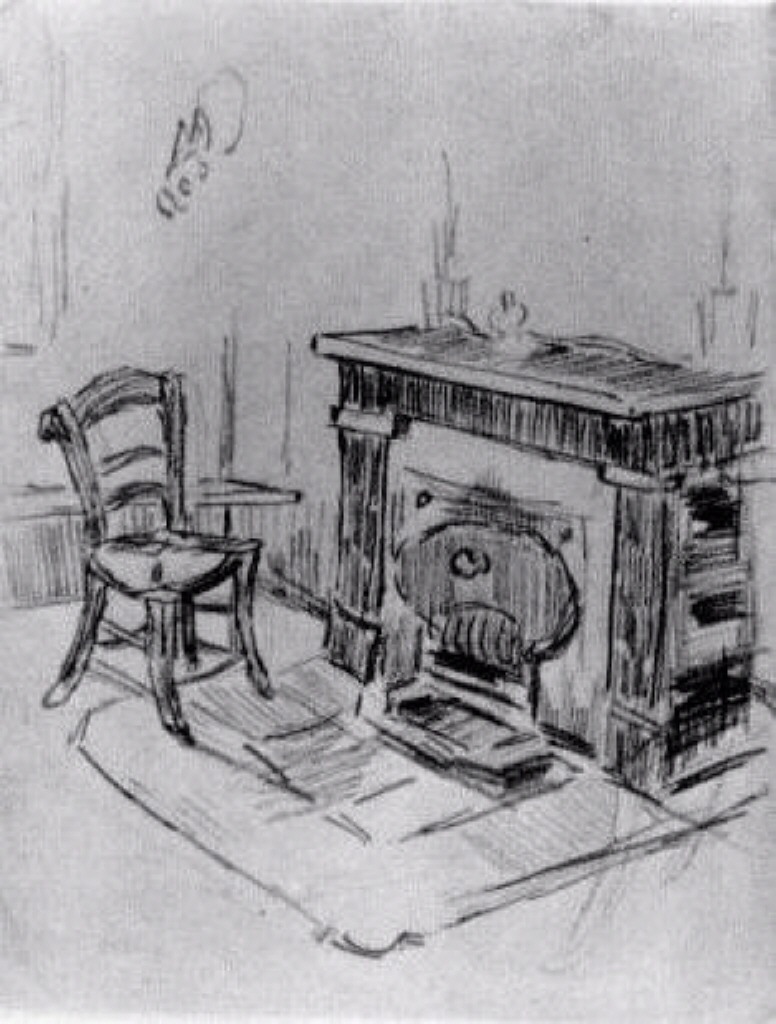The drawing depicts an old-fashioned room with a black and white, possibly charcoal-rendered, scene. Dominating the center-right of the image is a fireplace or iron stove, identifiable by its circular or oval entrance and accompanying grate. The fireplace sits incongruously atop a rug, which features some black detailing, hinting at possible unsafe placement. The room's background is shaded in gray tones, contrasting against the monochromatic elements. To the left of the fireplace is a wooden chair, distinctive by its lack of armrests and simplistic, vintage design. Above the fireplace, on the mantle, sit two plants, each in a container, adding a hint of life to the otherwise sparse setting. The room overall feels quaint and old-fashioned, with its grayish-white walls and slightly darker floor, enhancing the antiquated style of the furnishings. There are no people or text present in the image, adding to its quiet and contemplative atmosphere.